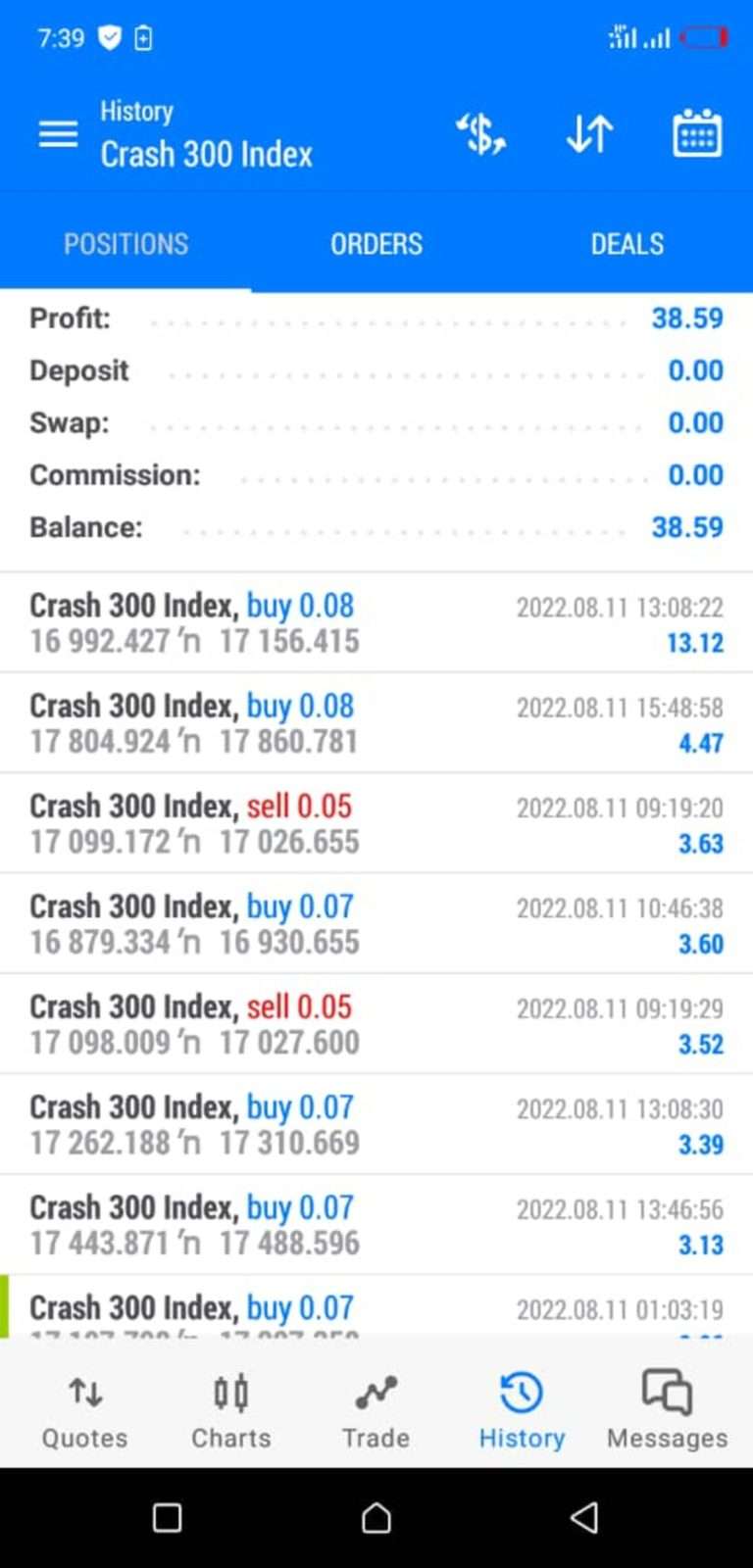This is a highly detailed screenshot from a smartphone or tablet screen, displaying a trading application interface at 7:39 (time not specified as AM or PM). 

At the top left corner, a white shield icon featuring a blue checkmark indicates some form of security status. Adjacent to it is a battery symbol with a plus sign, suggesting that the battery needs charging; its icon is highlighted in red due to low battery. The dual SIM functionality of the device is evident from two sets of cell phone signal bars on the right-hand side of the status bar. Both data indicators are full, situated on the left.

Underneath, on the left, are three horizontal lines representing the menu or settings. Next to this in bold white text is "History" followed by "Crash 300 Index." There are arrows pointing left and right, accompanied by a dollar sign, an up and down arrow, and a calendar icon.

The main section displays several menus where "Business" is selected, indicated by a grayish-blue background and a white underline. The unselected options include "Orders" and "Deals."

In the detailed white section, on the left is black text, and on the right is dark blue text starting with:

- Profit: $38.59
- Deposits: $0
- Swap: $0
- Commission: $0
- Balance: $38.59

Continuing with transaction details:
- "Crash 300 Index, Buy $0.08" in cyan blue.
- Additional details in gray text: $16, $992.427, hash n $17, $156.415.
- Timing details in gray on the right: $20.22.08.11, $13.08.22 (military time), and in blue $13.12.

Further transaction entries include:
- "Sell $0.05" in red for $3.63.
- "Buy $0.07" for $3.60.
- "Sell $0.05" for $3.52.
- "Buy $0.07" for $3.39.
- Another "Buy $0.07" for $3.13, with additional texts cut off.

At the bottom, the interface features tabs such as "Quotes" with an up and down arrow, "Charts" with stacked rectangles, "Trade" with a graph symbol, "History" (current selection) with a clock face and circulating arrow, and "Messages" represented by two chat bubbles. The device's lower bezel includes standard navigation buttons: a square (apps overview), a home button, and a back arrow.